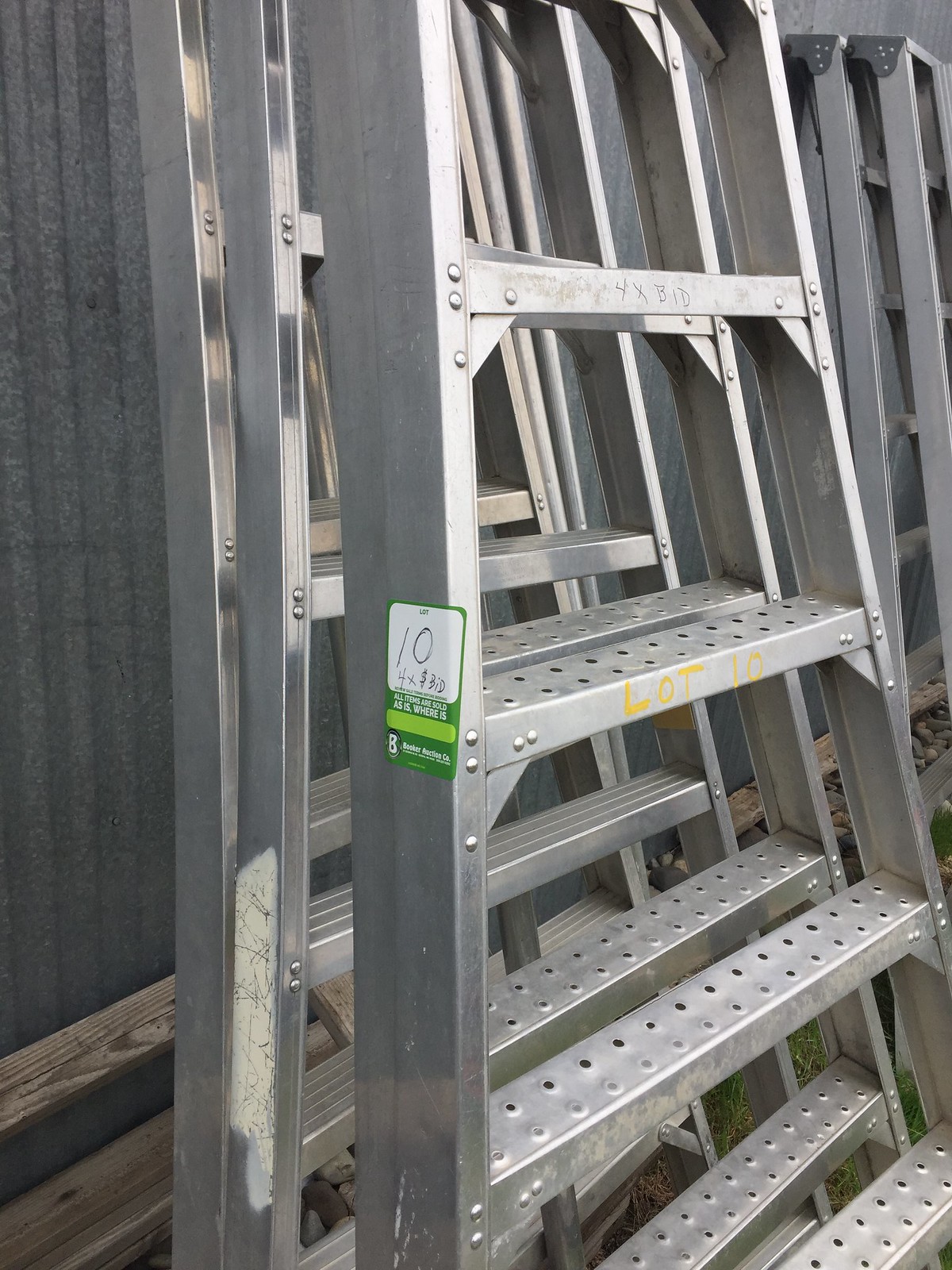This is a vertical, color photograph of a silver, metal (possibly aluminum or stainless steel) extension ladder. The ladder appears to be in a folded position and is leaning against a gray wall adorned with vertical stripes and perpendicular wooden strips. The ladder features steps with black holes for traction. Notably, a white and green sticker on the ladder displays the numbers "10 x 4 x 30" though some text is illegible. Additionally, the front of the ladder has orange lettering that reads "Lot 10." In the background, slightly to the top right, there are more stacked ladders, suggesting a storage area for ladders. The scene is filled with an industrial atmosphere, emphasized by the presence of multiple ladders and the structured background elements.